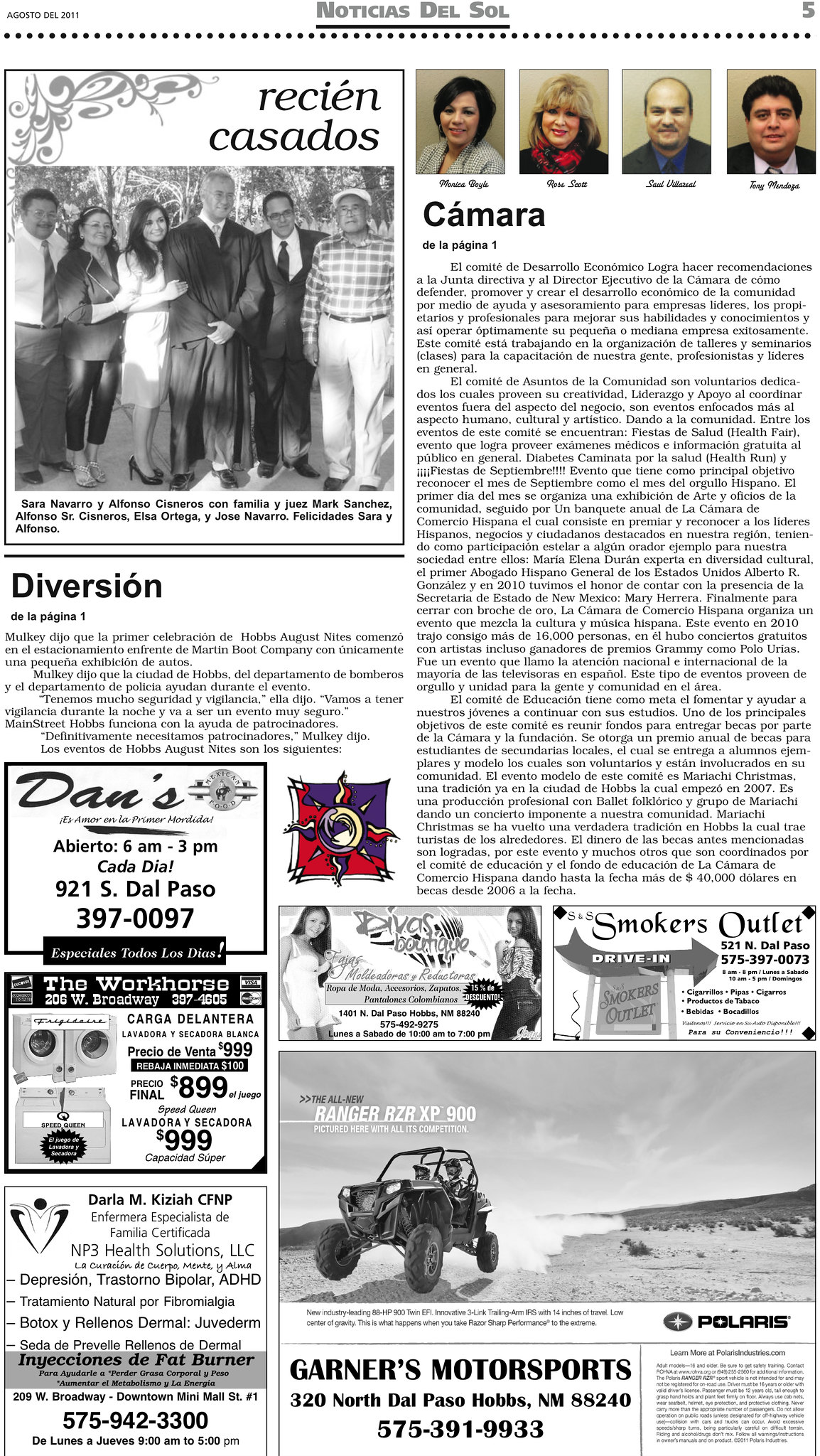The image is a digital screenshot of a magazine page, potentially from a newspaper as well. The main header reads "Noticias del Sol," indicating that the text is in Spanish. Prominently, there is a photo of a large group of people, with the central figure wearing a very large black gown, suggesting a graduation, and the words "Recién Casados" are visible. In the top-right section of the page, there's a row of four smaller photos featuring two women and two men, labeled with the word "Camara" beneath them. Below these images is a lengthy article in Spanish, the text of which is too small to read. To the left of this editorial section is another black and white photograph of five or six people, including someone appearing to wear a graduation cap and gown. Additionally, there are various advertisements scattered throughout the page. On the bottom left is an ad for "Dan's," while on the bottom right, there’s an ad for "Smokers Outlet Drive-In." Just below that is a buggy or ATV advertisement by Polaris for the "Ranger RZR XP900," associated with Garner Motorsports. Other notable ads include ones labeled "Devos" displaying two women and one titled "Diversion."